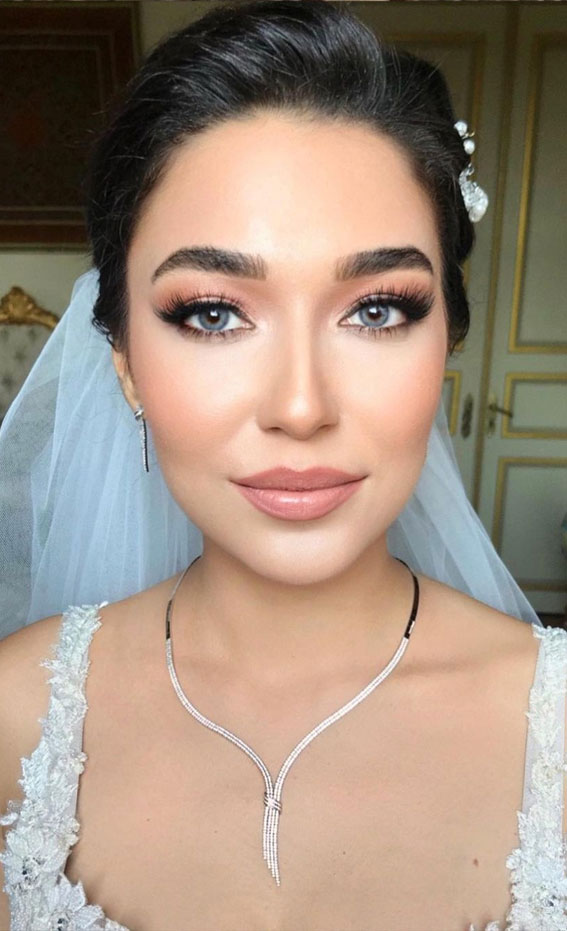This close-up photograph captures a bride in meticulous detail. Her dark black hair is elegantly tied up, adorned with two white pearls and a crystal ornament on the left side, and her veil, a delicate white lace, is attached at the back of her head. Her makeup is exquisitely done, featuring thick, luscious black eyelashes, enhanced dark eyebrows, and blush-colored eyeshadow. Her gray eyes, framed by both upper and lower lashes treated with mascara and eyeliner, convey a captivating look. She has a pale complexion with a hint of blush on her cheeks and rose-colored lips that look dewy.

She wears a stunning diamond choker necklace, shimmering with small diamonds and silver accents, which matches her dangling silver earrings. Her dress, glimpsed from just above the breasts upward, is sleeveless and adorned with ornate silver floral lace and appliqué. The elegant outfit is complemented by the sophisticated backdrop, which resembles a royal castle setting, with off-white, gold-trimmed walls. A white cushioned chair with gilded edges and a muted picture frame on the wall add to the luxurious ambiance. This detailed portrayal perfectly encapsulates the beauty and elegance of the bride on her special day.